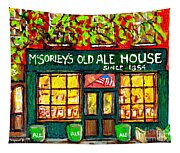The image is a detailed color illustration in a painterly style, depicting the front elevation of McSorley's Old Ale House. The scene is rendered in vibrant shades of red, green, black, white, and yellow, emphasizing various elements of the historic establishment. The building's prominent green facade features double doors with glass tops and a green border on the sides, adorned with white lettering that reads "McSorley's Old Ale House" and "Since 1854" painted above. An American flag flutters above the entrance, adding a patriotic touch. Below the signage is a pink mural, and at street level, the illustration shows green barrels labeled "Ale" in white text lined up on the sidewalk. There is evidence of graffiti-like patterns, especially above the door, adding a modern urban feel to the historic site. Flanking the doors are windows with nine panes each, through which soft interior lighting can be seen. The upper portion of the image reveals a larger red building with balconies and numerous windows partially obscured by overhanging tree branches. This landscape-oriented illustration captures both the charm and vibrancy of the old ale house as viewed from the street.